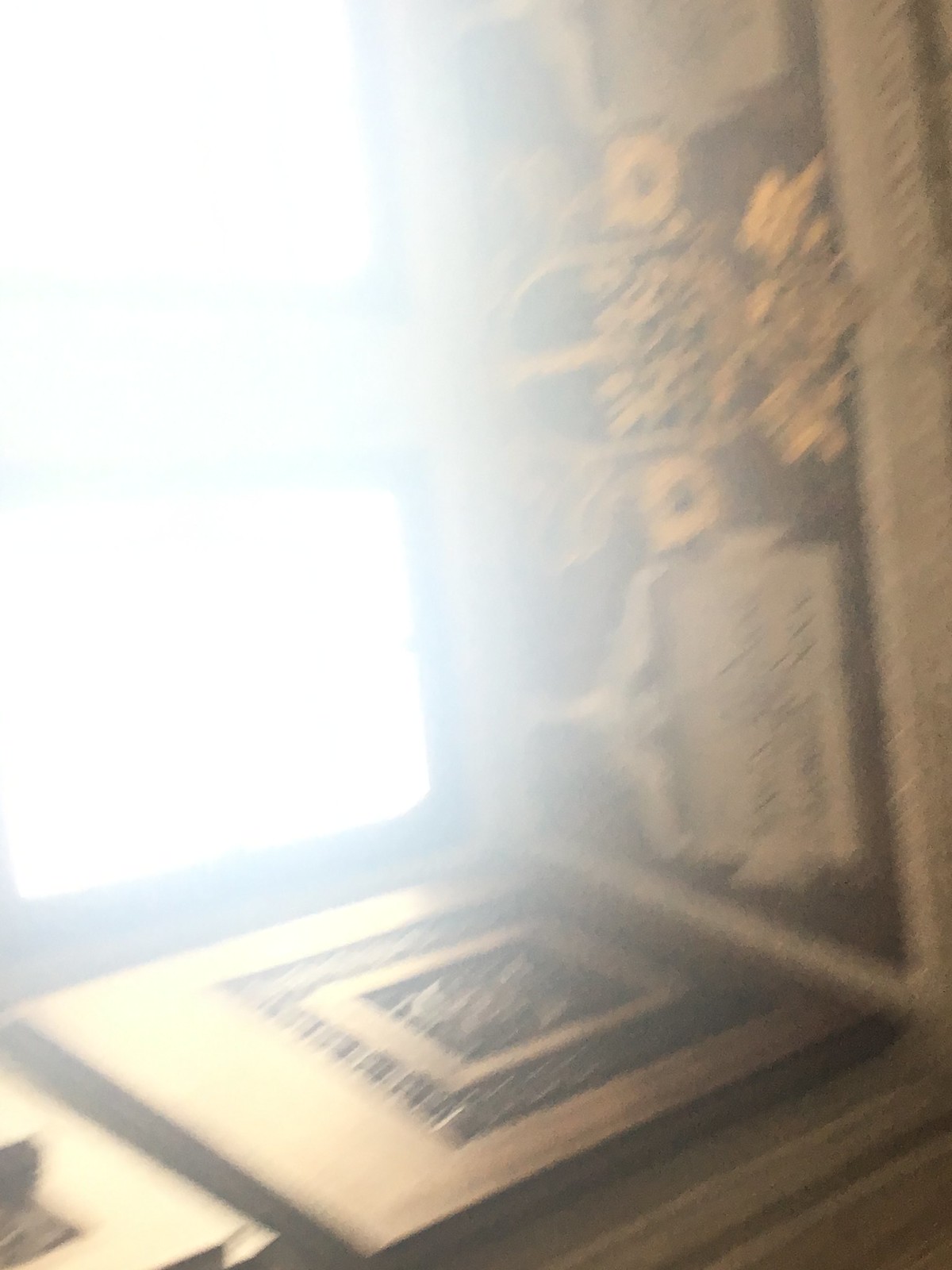The image is an indistinct, vertically oriented photograph, approximately 50% taller than it is wide. The central feature is a window in the upper left-hand corner that extends down roughly two-thirds of the image and spans about 40% across. This window is allowing a substantial amount of light, possibly sunlight, to pour in, creating a significant glare that washes out much of the image. The photograph is notably blurry, making it difficult to discern specific details clearly. 

Inside the windowsill area, there appears to be a horizontally laid tapestry on the right-hand side. On the left side of the windowsill, there's an abstract representation of a pot and another on the right, flanking what could be interpreted as a face in the middle. These objects seem to be drawn in light brown on a dark brown background. Beneath these, there's a picture frame located at the bottom portion of the windowsill. Owing to the bright light and blur, it's hard to tell more about the scene or any potential texts, dates, or locations of the photo, although it clearly seems to be taken indoors.